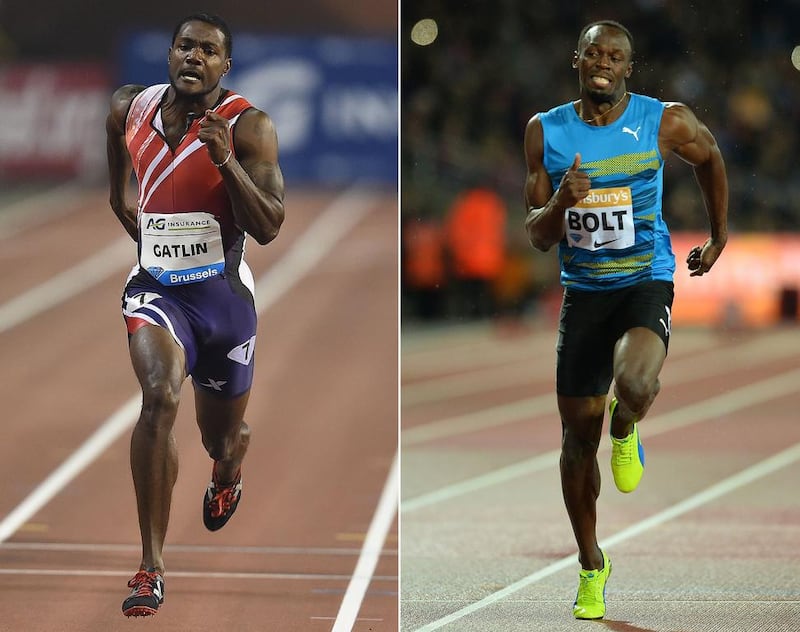The image features side-by-side pictures of two professional track and field runners known for competing in the 100-yard dash. The runner on the right is the renowned Usain Bolt, a black man with short black hair. He is adorned with a gold necklace and wears a blue, sleeveless Puma jersey with "Bolt" written in black on a sticker, which also displays the Nike logo on his stomach. Bolt has on black running shorts and neon yellow track shoes embellished with a blue Puma logo. Captured in motion, Bolt appears to be sprinting, his left knee lifted as he runs on a darker brown lane track lined with white separators.

To the left is another runner identified as Gatlin. He is wearing a red one-piece running suit with cut-off sleeves. The name "Gatlin" is seen in black text on a sticker positioned on his stomach area. His outfit includes dark purple running shorts and black shoes with red laces. Gatlin, too, is captured mid-sprint, mirroring Bolt's active running pose. Both athletes are photographed on their respective lanes of a professional track.